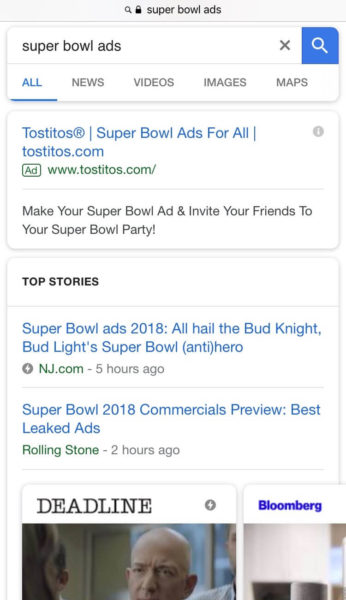A detailed caption for the screenshot could be:

"Screenshot of a Google search results page for 'Super Bowl ads.' At the top of the page, there is a search icon and a lock. The search term 'Super Bowl ads' is displayed in a white rectangular box in a larger font. Below it, there are tabs labeled 'All,' 'News,' 'Videos,' 'Images,' and 'Maps,' with 'All' selected and highlighted in blue.

The first search result is an advertisement from Tostitos, with the headline 'Tostitos Super Bowl Ads for All - Tostitos.com,' and a green URL 'www.tostitos.com.' The ad's description reads, 'Make your Super Bowl ad and invite your friends to your Super Bowl party.'

Beneath this, a banner labeled 'Top stories' displays two articles. The first, from NJ.com five hours ago, titled 'Super Bowl ads 2018: All hail the Bud Knight, Bud Light’s Super Bowl antihero.' The second article, from Rolling Stone two hours ago, is titled 'Super Bowl 2018 commercials preview: Best leaked ads.' Both time stamps are in gray.

Below these articles are two cut-off images: the first showing part of the 'Deadline' logo with a glimpse of a couple of people, and the second one with partial text from 'Bloomberg,' which appears mostly blank with some black content.

The visual layout emphasizes the immediacy and variety of information available on the topic of Super Bowl ads."